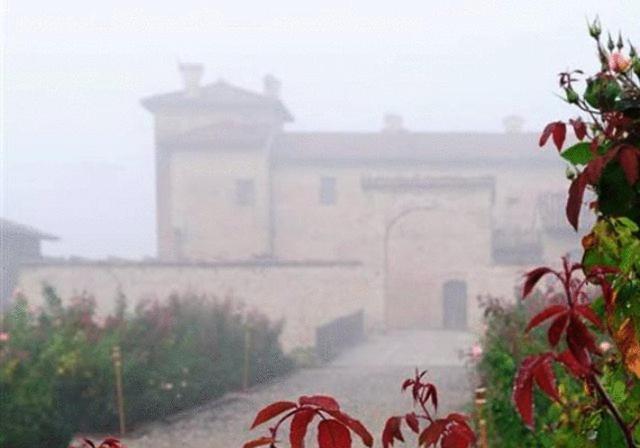This is a horizontally aligned, rectangular image that appears somewhat blurry, as though taken through a window or in foggy conditions. The focal point is a stone building with a rectangular shape made of yellow-tan bricks and topped with a brown roof. The building features an arched stone entrance and is reminiscent of an older European architectural style. The sky behind the building is partly cloudy, with patches of blue and light gray-white clouds.

A prominent stone walkway leads up to the building, flanked on both sides by gold-colored posts and lush vegetation. On the left side of this walkway, tall green bushes with red-tipped leaves rise up, while on the right side, a close-up of green leaves intermixed with dark red ones is visible. Additionally, a guard rail can be seen on the left side of the walkway, enhancing the sense of structure and path.

In the foreground, a garden featuring more green and red-leaved bushes is evident, particularly concentrated at the bottom right of the image. The overall atmosphere suggests a quiet, possibly early morning scene, captured during the day. The combination of the foggy ambiance and the soft cloud coverage gives the picture a serene and muted quality.